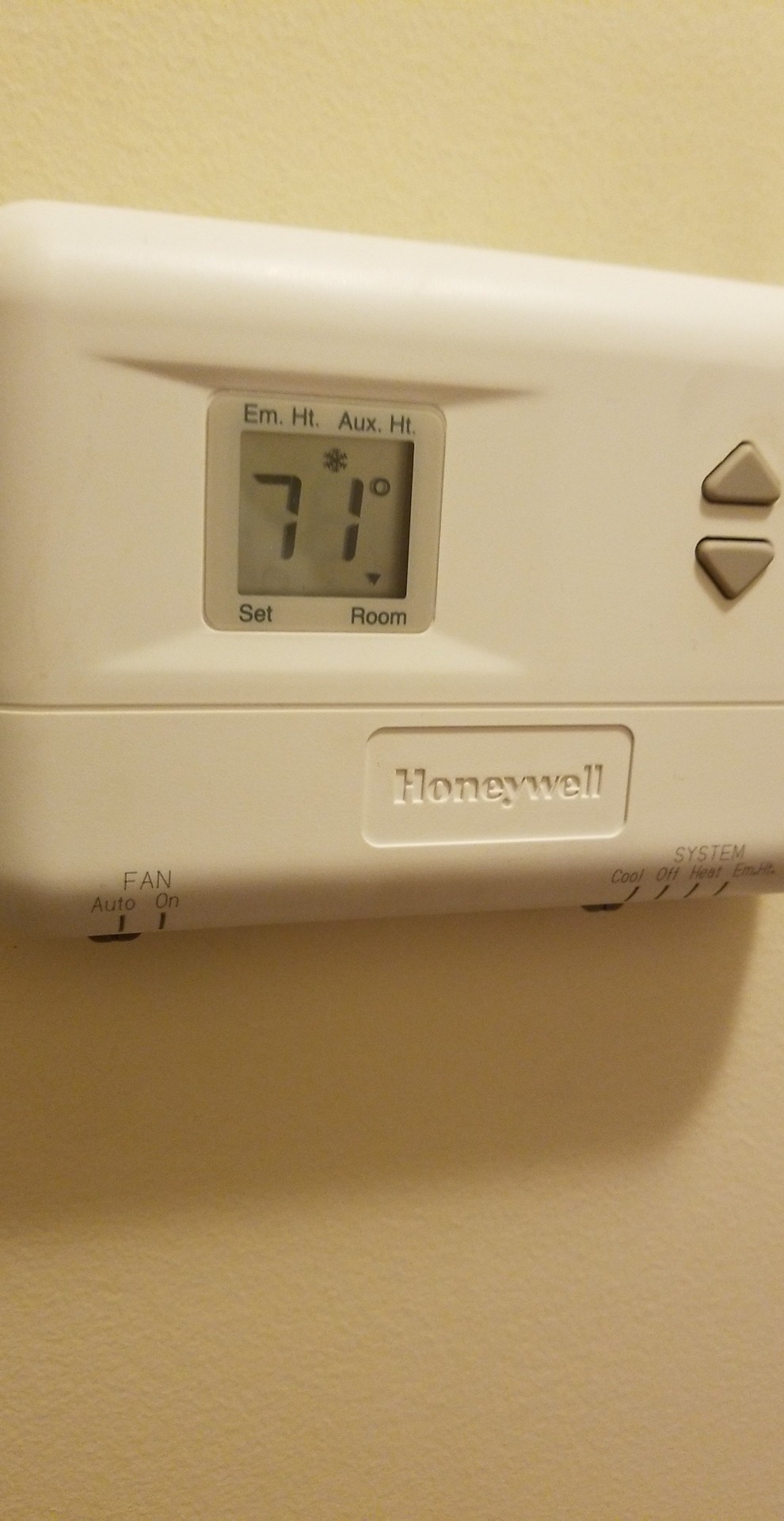The image displays an off-white Honeywell thermostat mounted on a yellow wall. The Honeywell name is inscribed on the front of the device, within an engraved rounded square at the bottom. On the left side of the thermostat, there are switches labeled "Fan," "Auto," and "On," each with corresponding black lines beneath. To the right, the switch functionality labeled "System" is accompanied by additional markings below. The device features two brown arrow buttons for adjusting settings, one for increasing and one for decreasing the temperature.

The digital display, encased in glass, shows a current temperature reading of 71 degrees. Above this reading, there is a small star symbol. The display also includes labels for "Set" on the left side and "Room" on the right side, both in black letters. At the top of the display area, the abbreviations "em.ht." and "aux.ht." can be seen, with a small black arrow pointing downwards just above the "Room" label, indicating that the 71-degree reading pertains to the room temperature.